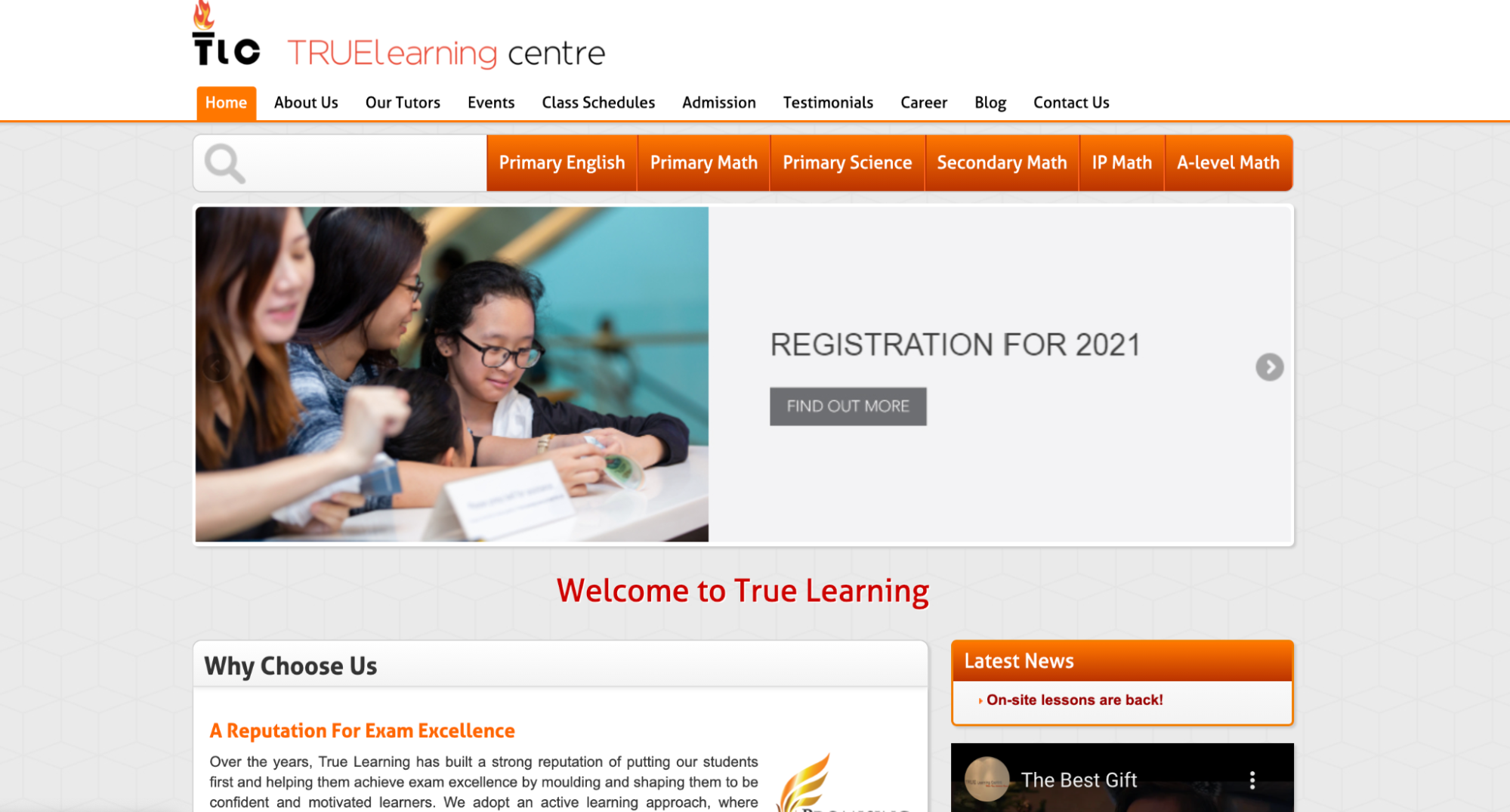Here is a cleaned-up and more detailed caption for the provided image description:

"This screenshot captures the homepage of the True Learning Center (TLC) website. The header displays the TLC logo in black, with a stylized 'T' topped with flames, resembling a torch. The full name, 'True Learning C-E-N-T-R-E,' highlights 'T-R-E-E' in all capitals and the 'L' in 'Learning' also capitalized.

The navigation menu at the top includes options such as Home, About Us, Our Tutors, Events, Class Schedules, Admission, Testimonials, Career, Blog, and Contact Us. The selected 'Home' tab is highlighted with an orange rectangle. A search bar with a magnifying glass icon is positioned nearby.

Below this, a series of orange rectangles feature the text for subject offerings: Primary English, Primary Math, Primary Science, Secondary Math, IP Math, and A-Level Math, all written in white.

A prominent gray rectangle announces registration for 2021 with a 'Find out more' call-to-action in white text.

The main body of the page displays a welcoming message in red: 'Welcome to True Learning.' Below this, the latest news section under 'Why Choose Us' touts the center’s reputation for exam excellence, stating that over the years, True Learning has built a strong reputation. Additional information is provided to support this claim."